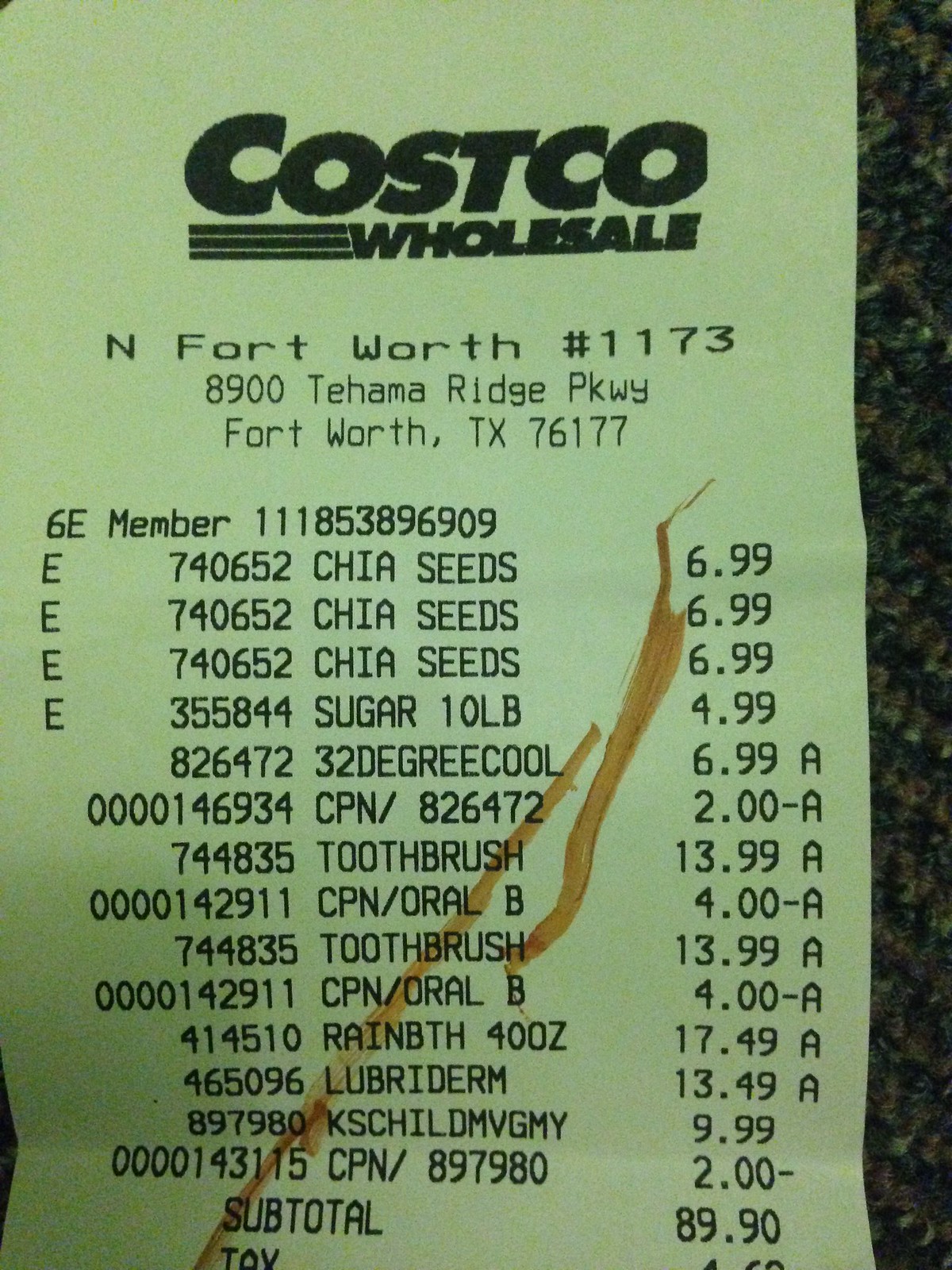In this detailed close-up photograph, the white Costco Wholesale receipt lies on a dark, granite or Formica tabletop. The receipt, slightly tinged with a muted green hue due to the lighting, prominently displays the store details at the top: Costco Wholesale, North Fort Worth, location number 1173, situated at 8900 Tahoma Ridge Parkway, Fort Worth, Texas 76177. The receipt lists various purchased items including three chia seeds priced at $6.99 each, a 10-pound bag of sugar for $4.99, an item labeled "32 Degree Cool" costing $6.99, several toothbrushes marked under different codes with prices of $13.99 each and applicable coupons reducing some prices by $4 each, a 40-ounce Rain Bath item for $17.49, and Lubriderm lotion priced at $13.49. There are also mentions of codes like CPN 826472 applying a $2 discount, and a KS child-related item costing $9.99 with a coupon reducing it by $2. The subtotal amounts to $89.90, followed by some tax information where the details become illegible. Notably, across the receipt from the bottom left to the upper right corner, there's a streak of reddish-brown stain that could be from blood, a marker, or coffee.